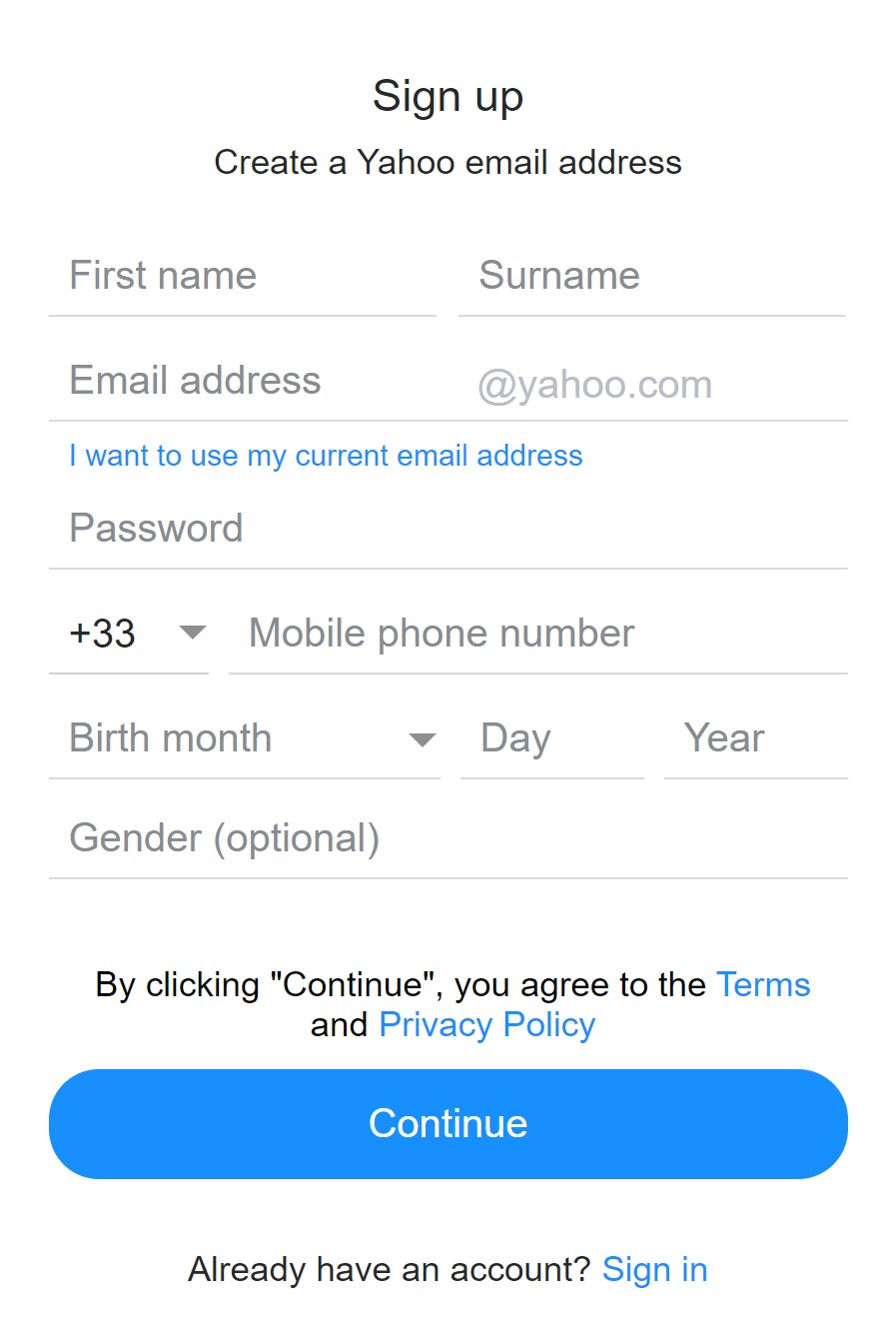This screenshot depicts the Yahoo sign-up page. At the top of the page, the heading "Sign Up" is prominently displayed. Below this, in black text, it states "Create a Yahoo Email Address." The form consists of several fields and options organized as follows:

1. **Personal Information:**
   - **First Name and Surname:** Two side-by-side fields for entering the first name and surname.

2. **Email Information:**
   - **Yahoo Email Address Field:** A single field for entering the desired email address ending with "@yahoo.com."
   - **Use Current Email Address:** A link in blue text allowing users to opt for their existing email address.

3. **Password:**
   - **Password Field:** A field for entering the chosen password.

4. **Contact Information:**
   - **Phone Number:** Begins with a drop-down menu defaulting to "+33" for the country code, followed by a field to enter the mobile phone number.

5. **Personal Details:**
   - **Birthday:** A section with three fields for birth month (a drop-down menu), day, and year.
   - **Gender (optional):** Field labeled "Gender" with the word "optional" in parentheses.

6. **Agreement to Terms:**
   - **Continue Prompt:** Text stating, "By clicking Continue, you agree to the Terms and Privacy Policy," with "Terms" and "Privacy Policy" being clickable links.
   - **Continue Button:** A prominent blue button labeled "Continue."

7. **Alternate Sign In:**
   - **Existing Account:** Text stating "I already have an account," followed by a clickable "Sign In" link.

The background of the page is white, providing a clean and straightforward design for ease of use.